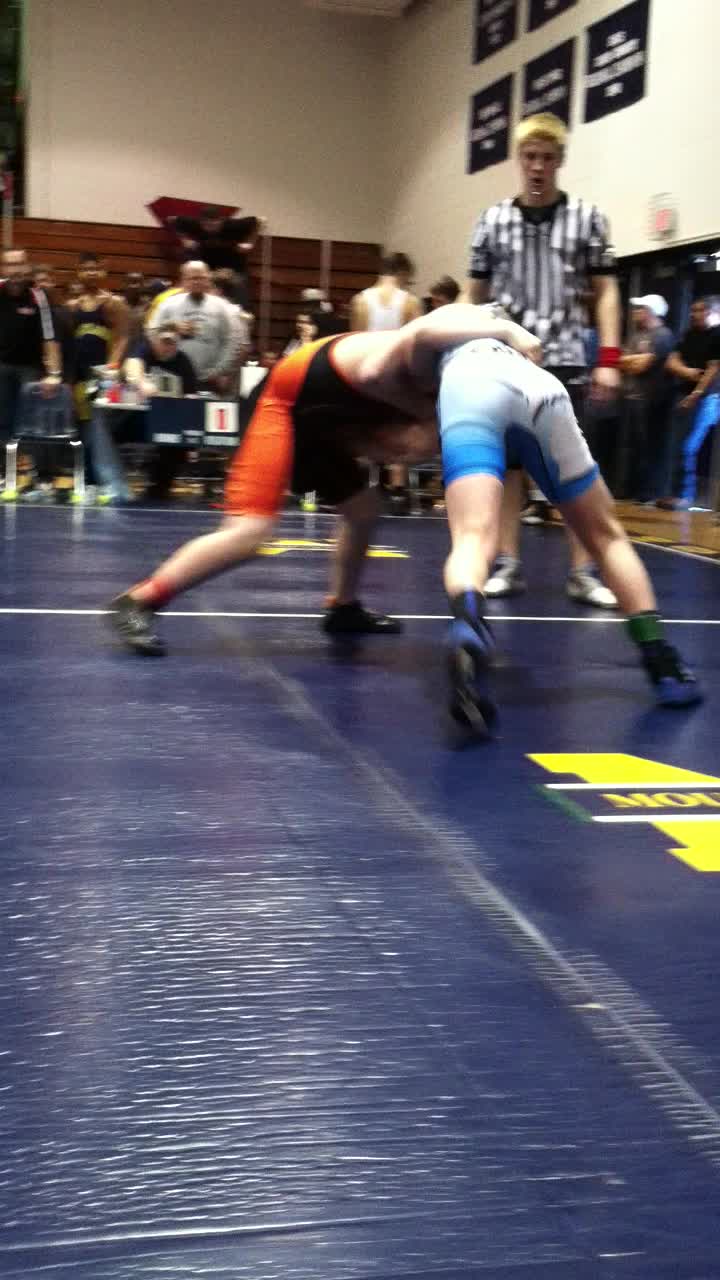This image captures a high school or college-level wrestling match taking place in a gymnasium. Two male wrestlers are engaged in a bout on a dark blue mat adorned with a partially visible yellow logo that reads "M-O-U." One wrestler is clad in a blue and white bodysuit, while the other sports an orange and black bodysuit. The wrestler in blue and white features distinctly patterned shorts that transition from white to varying shades of blue, along with black shoes and socks. The opponent in the orange and black attire has a predominantly black front with orange detailing on the back and legs, complemented by orange socks and black shoes.

A referee, dressed in a black and white striped shirt and sporting blondish-brown hair, stands nearby with a whistle in his mouth and a red wristband visible. In the background, a group of spectators—likely coaches and fellow team members—watches intently. The scene exudes the vibrant energy of a school gymnasium during a competitive wrestling event.